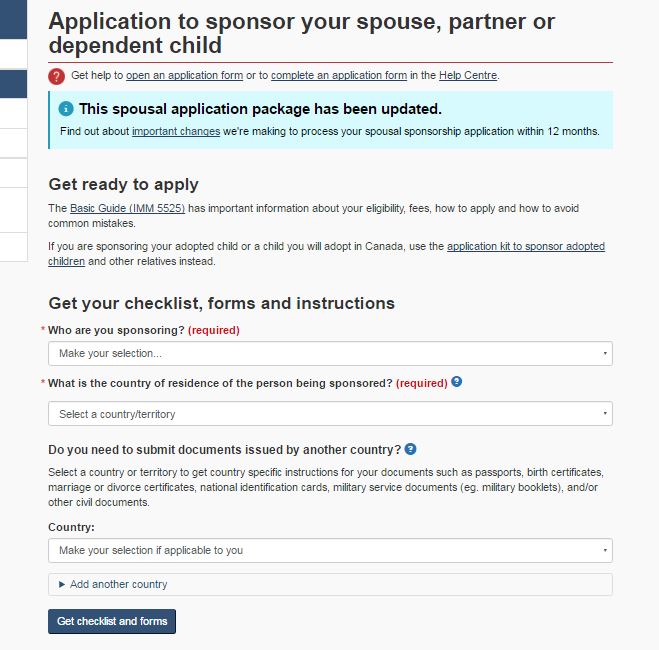"Screenshot Depicting the Sponsorship Application Process for Spouses, Partners, or Dependent Children from an Unknown Web Page: 

The top section of the page prominently features the title, 'Application to Sponsor Your Spouse, Partner, or Dependent Child.' Below it, a prompt invites users to seek assistance in either opening or completing the application form via the Help Center.

A conspicuous turquoise banner indicates that the spousal application package has been updated, urging users to discover essential changes aimed at processing applications within a 12-month timeframe. Prospective applicants are encouraged to prepare their submissions by consulting the basic guide, IMM5525, which contains crucial information about eligibility, fees, application procedures, and advice on avoiding frequent mistakes.

The guidance further clarifies that individuals sponsoring adopted children or children they plan to adopt in Canada should use a different application kit tailored to sponsoring adopted children and other relatives.

The webpage continues with a series of required fields where applicants must specify the individuals they are sponsoring and the country of residence of the person being sponsored. It includes dropdown menus for selecting countries or territories to obtain country-specific instructions for necessary documents such as passports, birth certificates, marriage or divorce certificates, national identification cards, military service documents, and other civil documents. An option to add documents from another country is also present.

At the bottom of the page, users can access checklists and forms pertinent to their application process.

This image contains no photographic elements."